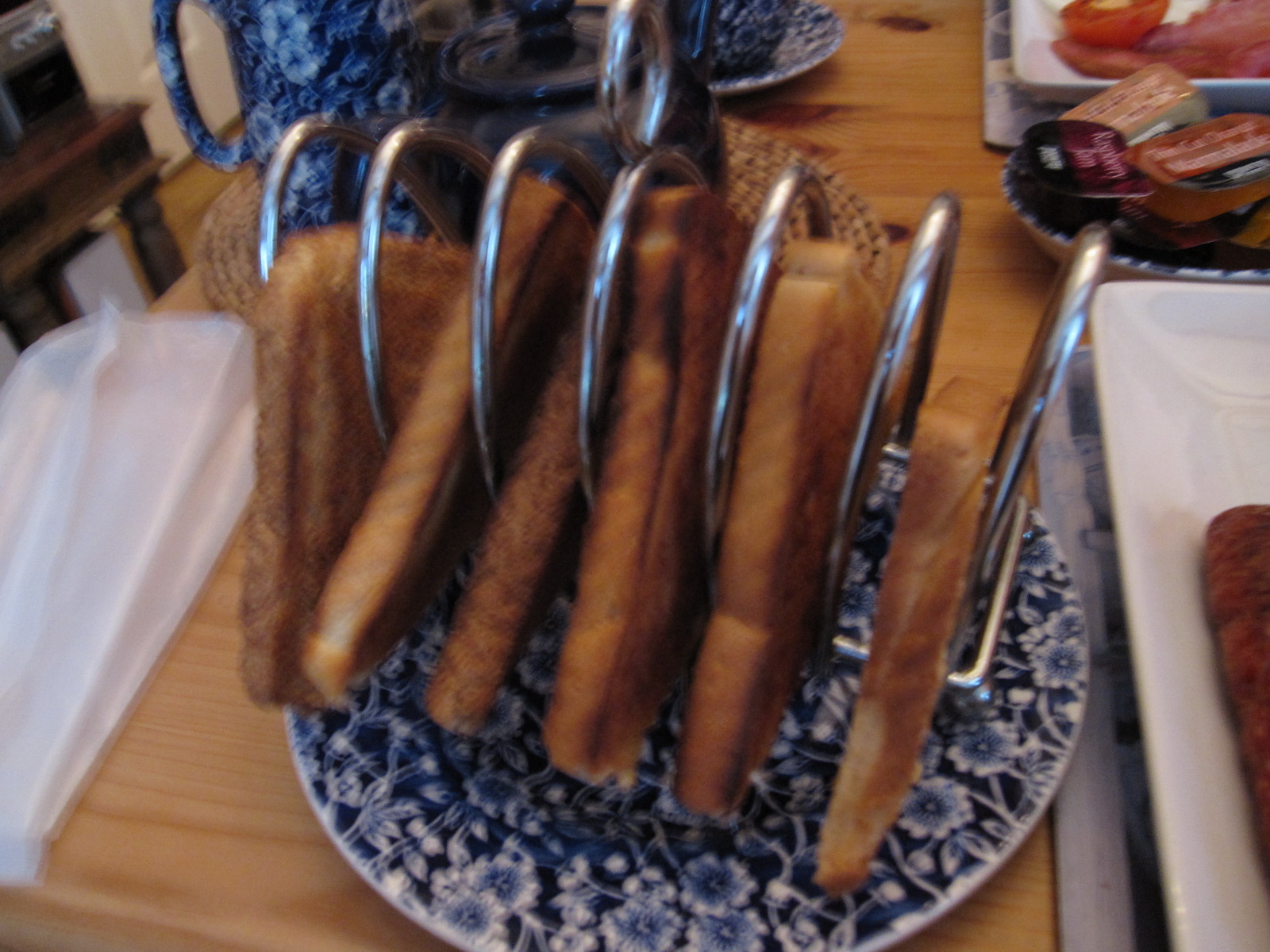The image captures an overhead, slightly out-of-focus photograph of a table setting, likely at a restaurant. The focal point is a silver toast rack holding six slices of diagonally cut, brownish toast halves. The toast rack sits atop a dark blue and white floral-patterned china plate. The table is made of light pine wood, displaying a distinct wood grain texture.

To the left and slightly behind the toast rack, there's a wicker bowl containing an indistinct, out-of-focus blue and floral item. Above and to the left, a small, off-focus desk with brown legs is partially visible in the top left corner, along with the corner of a white door nearby.

Adjacent to the toast rack on the right is a white dish, potentially holding a pastry, and further up, a white plate holding a blue bowl filled with dipping sauce. In the top right corner, a white dish with fried tomatoes and bacon is visible, accompanied by pre-packed jams on another matching blue and white dish. Additional tableware, including a cup and saucer, is subtly present in the background.